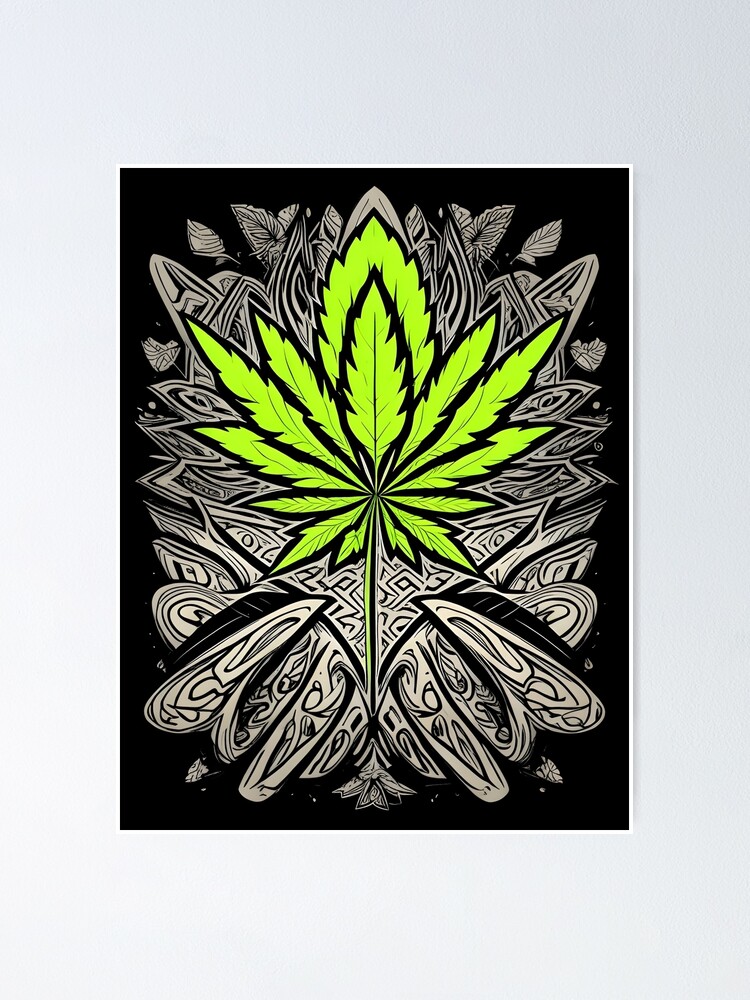The image is a digital artwork centered around a prominent green marijuana leaf with a thin stalk. The leaf has a black outline and is composed of 13 serrated points— six on each side and one in the center, which is the largest. This focal leaf is layered over an intricate background consisting of white and black abstract patterns, including geometric shapes and tribal designs, which create a sense of movement and depth. The background has three main layers: the base is an off-white or light gray, followed by a black layer, and the outer corners blend into a darker black. The dominant colors are green, black, and an off-white/gray shade, with the black and white patterns subtly enhancing the composition without any text in the image.